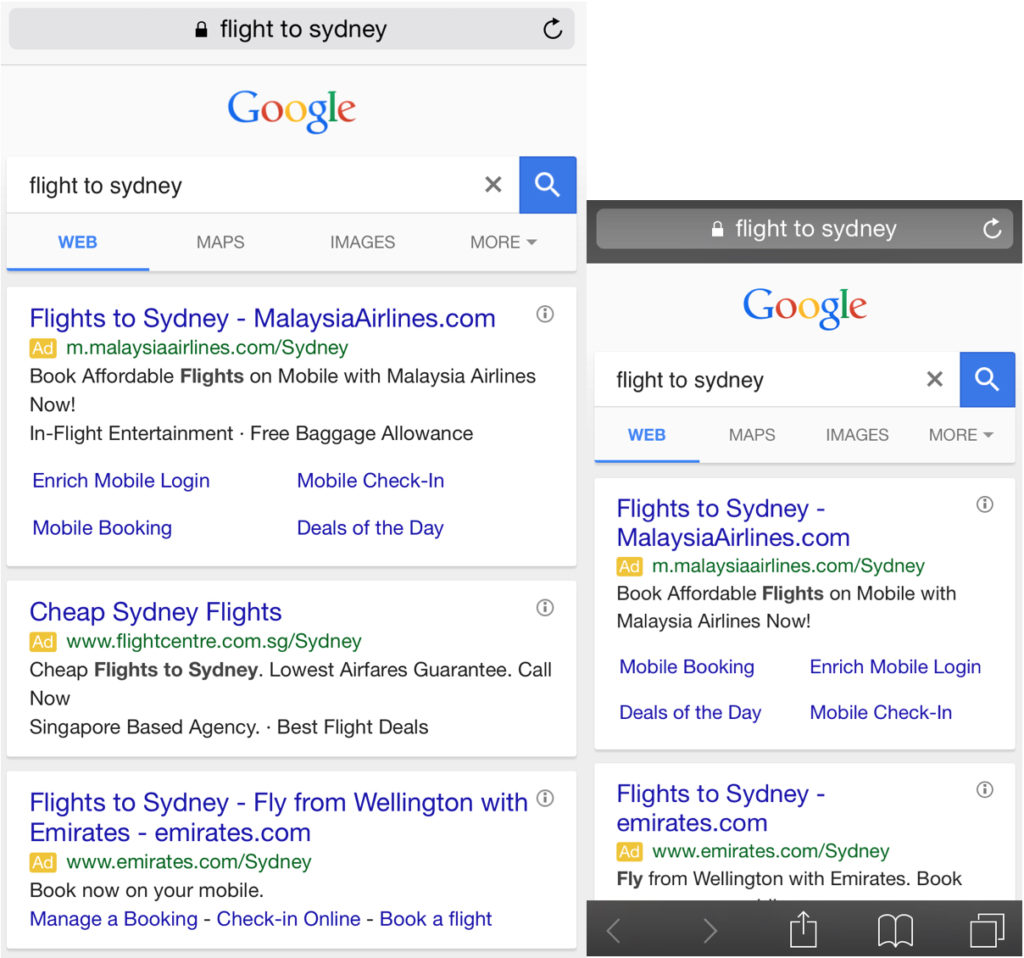"Discover affordable flights to Sydney, Australia, including deals from Malaysian Airlines and Emirates, departing from Wellington. Research options through Google Maps and web searches to find the best prices and routes. Utilize cognitive tools for detailed planning, measure distance with map views, and plot travel frequency using directional maps. Prepare for directional changes using cognitive devices and explore the best ways to travel between destinations. Verify travel information by checking books or online resources to ensure a smooth journey. Visualize the journey using horizontal and vertical measurement axes, and coordinate with conductors or travel guides for an organized trip plan."